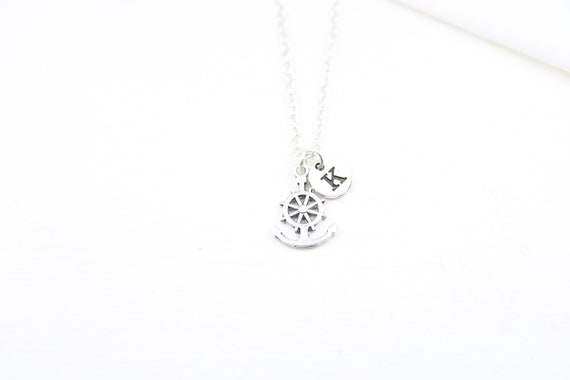The photograph features a silver necklace set against a predominantly white background, making it blend somewhat into its pale surroundings. The necklace comprises two distinct pendants. The larger pendant at the bottom features a detailed sculpture of an anchor integrated with a boat's steering wheel. Above it, the smaller pendant resembles a round coin, imprinted with the letter "K" in black. Despite the low resolution and slight blurriness of the image, the craftsmanship of the silver jewelry is apparent through the intricate design of the nautical-themed pendants and the clarity of the monogrammed coin.